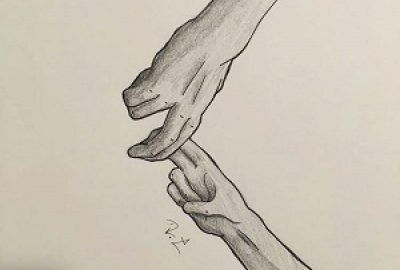This detailed pencil or charcoal drawing, likely created by a beginner artist, depicts two interlocking hands against an off-white or slightly grayish paper background. The adult hand, emerging from the top right of the image, has its thumb closed and the pinky and ring fingers curled, while the index and middle fingers interlock with those of a child's hand. The child's hand comes from the bottom left, its thumb closed over the last two fingers, and its palm visible, mirroring the grip with its first two fingers. The drawing captures the hands extending from the wrists without revealing much of the forearms. The shading adds a darker tone to the lower parts of the hands. An artist's signature, which appears to be in cursive and could be the initials "RT" or "RL," is situated beneath the bottom hand.